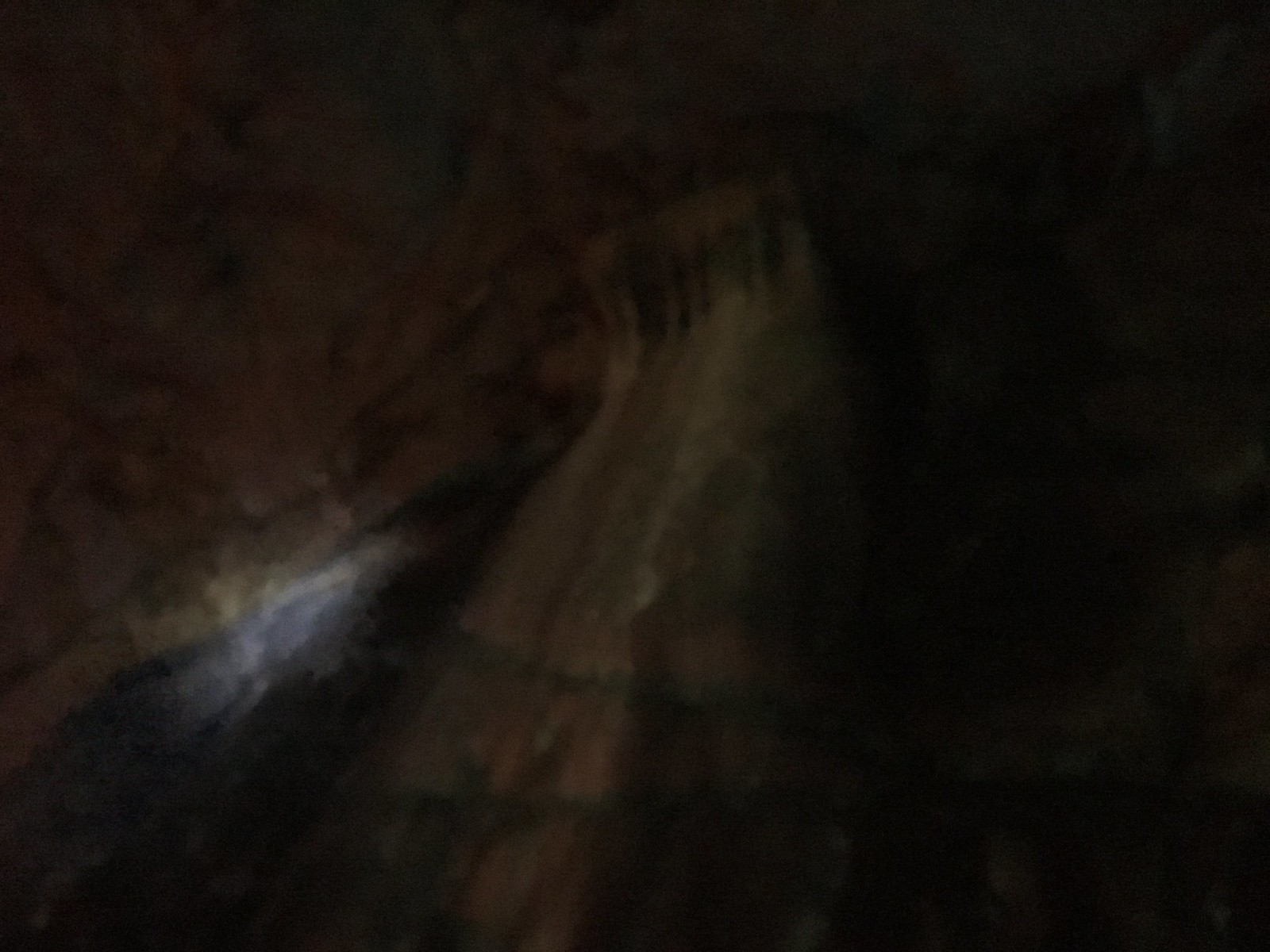The image portrays a dark, atmospheric scene reminiscent of a painting. The dominant colors are deep browns and blacks, creating a shadowy, almost mysterious ambiance. The composition appears to be the exterior of a cave, with the rocky surface enveloping the entrance, which is dimly lit, possibly by moonlight. The rocks are discernible above and around the cave opening, bathed in a faint light that contrasts with the encroaching darkness. Inside the cave, the interior is shrouded in blackness, except for a sliver of white light right at the threshold, hinting at some presence or object just inside. The front of the cave entrance is subtly illuminated, standing out against the indistinct, pitch-black backdrop that seems to blend into the night.